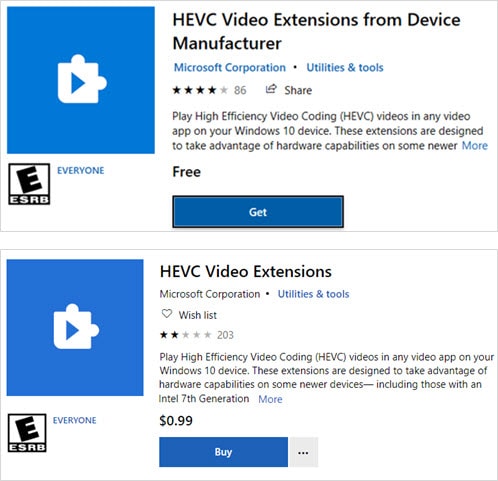This image captures a section of a sales webpage for Microsoft Corporation, specialized in offering add-ons for Windows devices. The page is designed with a minimalist aesthetic, featuring two distinct options for product extensions, each enclosed in thinly outlined rectangles that appear either gray or light blue.

Within each outlined rectangle, on the left-hand side, there is a prominent blue box adorned with an icon representing the specific extension available for purchase. Accompanying these icons is a rating indicator. The rating is displayed inside a black-outlined box, featuring an eye-catching large black 'E' that is slightly tilted. Beneath this 'E', in white letters, the text 'ESRB' is clearly visible, signifying that these extensions are rated 'Everyone' by the Entertainment Software Rating Board, indicating no purchase restrictions based on content.

The first rectangular option at the top of the page is promoting a video extension provided by the device manufacturer. This visually structured setup ensures customers can easily identify and select extensions suitable for enhancing their Windows experience without any age or content limitations.